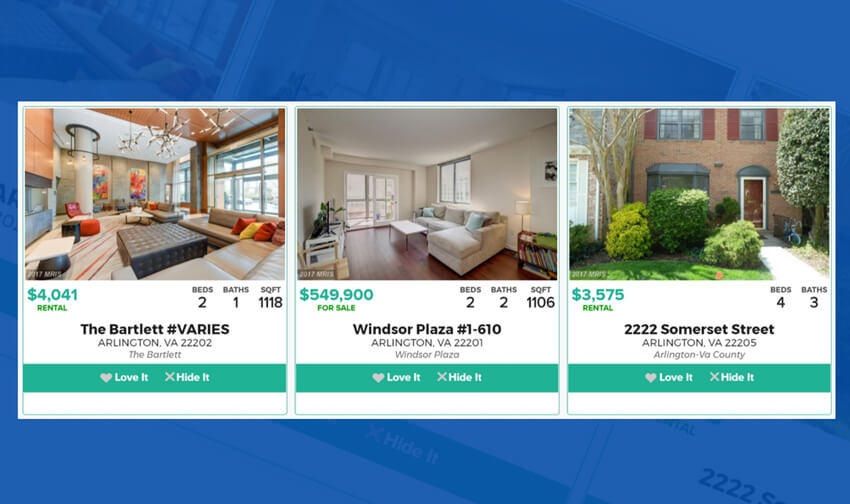The image features a blue background with faint, non-solid elements, suggesting part of a home setting. On the left side of the image, a couch is visible, while the right side reveals the upper section of a walkway, including a white ceiling. The image includes three rectangular sections with property details:

1. **Section One:**
   - **Image Description:** It depicts the entrance of a building featuring a large gray ottoman.
   - **Text Details:**
     - **Price:** $4,041 (highlighted in green)
     - **Type:** Rental
     - **Specifications:** 2 beds, 1 bath, 1,118 SQFT
     - **Property Name:** The Bartlett
     - **Location:** #Rarities, Bartletton, VA 22202

2. **Section Two:**
   - **Image Description:** Shows a white room with an off-white sectional sofa.
   - **Text Details:**
     - **Price:** $4,990 (highlighted in green)
     - **Type:** For Sale
     - **Specifications:** 2 beds, 2 baths, 1,106 SQFT
     - **Property Name:** Windsor Plaza
     - **Location:** #1610, Arlington, VA 22202

3. **Section Three:**
   - **Image Description:** Features the front view of a round townhouse.
   - **Text Details:**
     - **Price:** $3,575 (highlighted in green)
     - **Type:** Rental
     - **Specifications:** 4 beds, 3 baths
     - **Location:** 2222 Somerset Street, Arlington, VA 22205, Arlington County